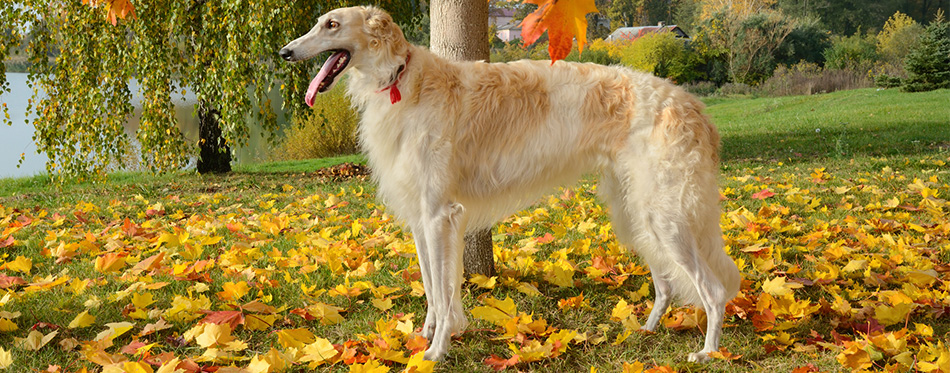In this picturesque autumn scene, a large, thin dog with a striking cream-colored coat adorned with light brown splotches stands prominently on a lush green lawn strewn with bright yellow and golden leaves freshly fallen from nearby trees. This dog, almost Great Dane-sized but of an indeterminable breed, boasts long legs and a pronounced pointy snout. With its mouth wide open and long tongue hanging out, the dog gazes intently to the left, possibly eyeing a pond situated in the distance. It wears a collar tinged with red and seems poised for either a swim in the nearby lake or simply catching its breath after a playful romp. Behind the dog, the scene is framed by trees, hinting at a serene park setting, with a backdrop of additional trees, patches of grass, and vague outlines of distant dwellings peeking through the foliage. The combination of green, orange, red, and blue hues contributes to the vivid, early-autumn ambiance of the landscape.